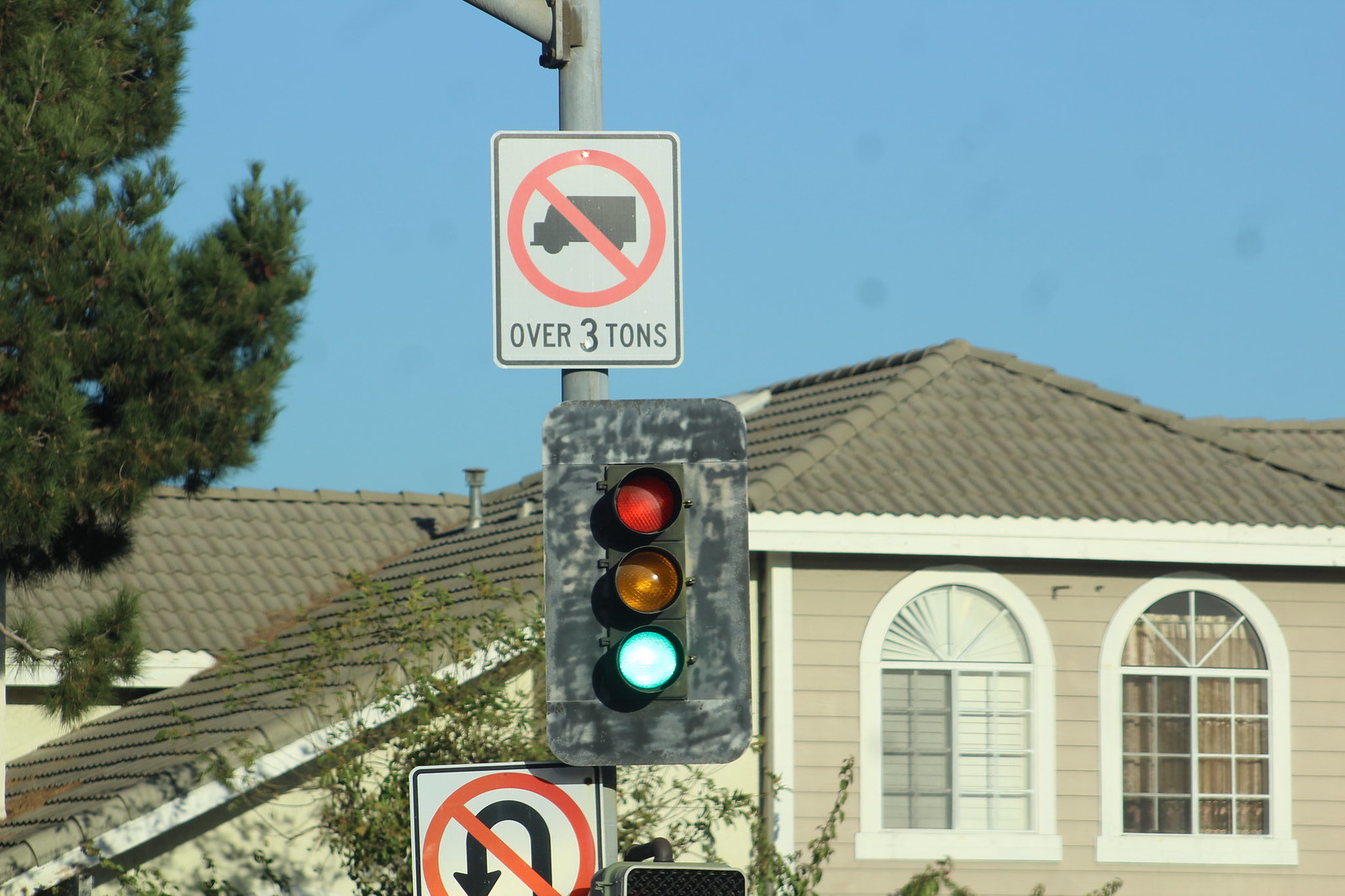The image depicts a traffic light mounted on a vertical pole with the green light currently illuminated. Below the traffic light, there is a no U-turn sign featuring a red circle with a bar across it. Above the traffic light, there's another sign prohibiting trucks over three tons, showing the silhouette of a truck with a red mark over it and the text "over 3 tons" underneath. Behind the traffic light is a gray, camouflage-like pattern. Additionally, a horizontal branch extends off-screen above this sign. On the left side of the image, part of a tree with ample green leaves is visible, as well as the right side of a house with light gray roof tiles and arched windows with curtains or blinds. The sky is clear and blue, indicating a cloudless day, and the overall setting appears to be in a residential area.